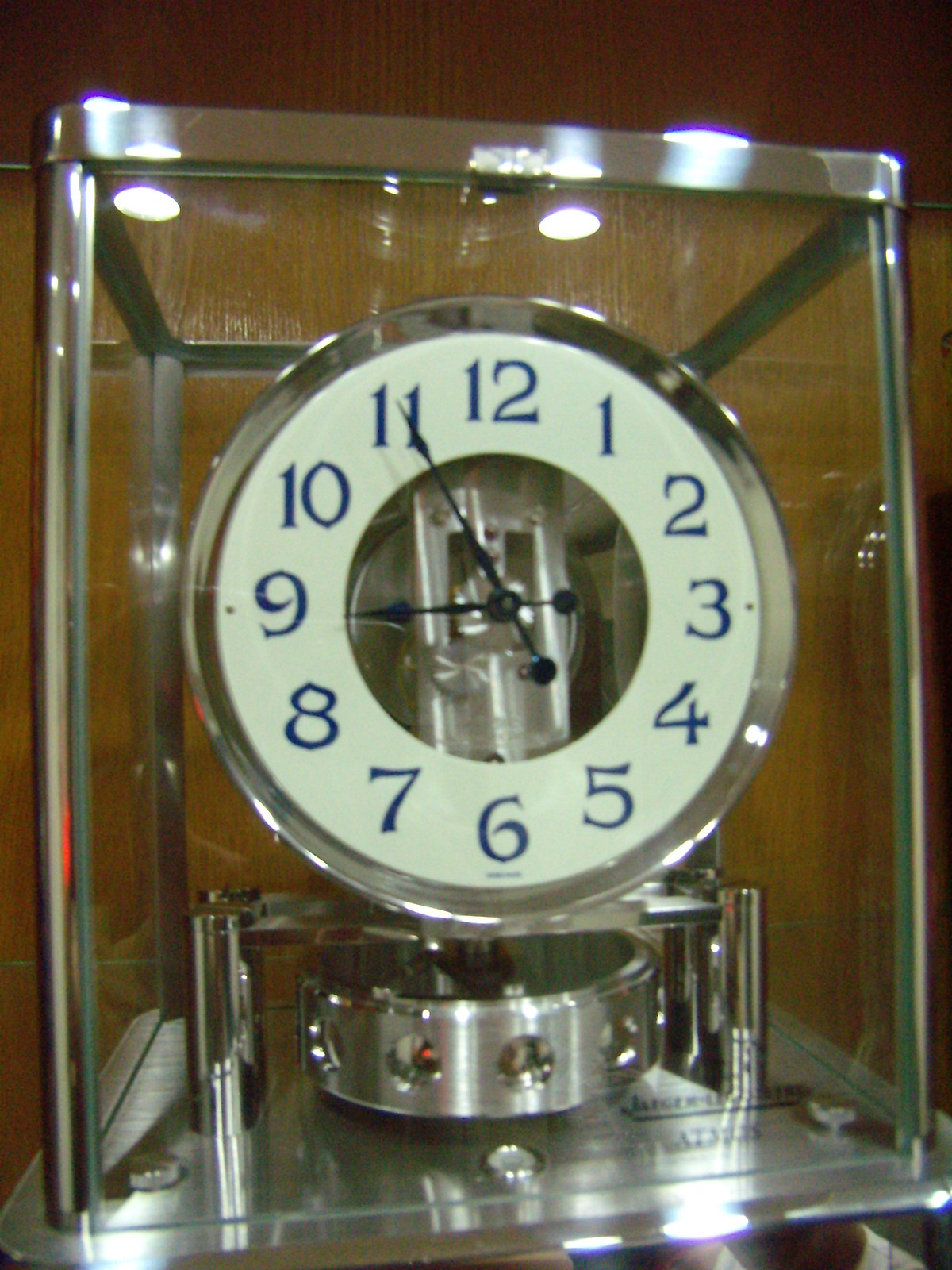The photograph features a close-up of a sophisticated clock encased in a rectangular glass box with a silver metal frame. The transparent glass body reveals the intricate mechanisms inside, including some visible metal pieces and cogs. Central to the clock is a round face with a creamy white background and a clear center cutout, through which the inner workings can be observed. The clock face is adorned with navy blue numbers from 1 to 12 and matching dark blue hands, giving it a sleek appearance.

The clock is mounted on a silver metal base supported by four small pillars. This structural platform seamlessly integrates the upper part of the clock with the base. Additionally, the base itself, which is silver and metallic, features some writing and appears to support a rotating circular disc beneath the clock. Reflections from an overhead light source can be seen glinting off the edges of the glass case, adding to the clock’s elegance.

The background of the image is a backdrop of dark brown wooden paneling, providing a warm contrast to the sleek, contemporary design of the clock.